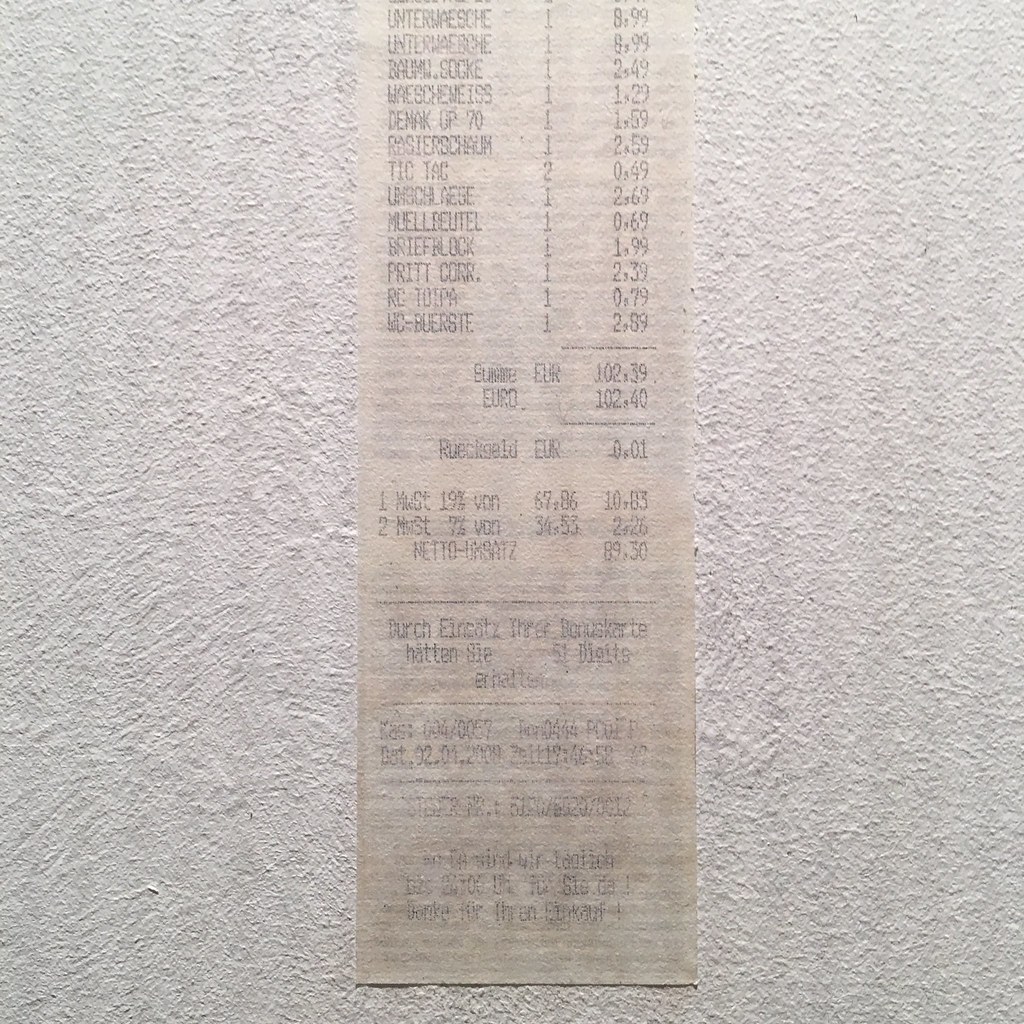This image captures a partial receipt printed on white paper with black text and numbers. The text on the receipt is faint, particularly towards the bottom where it becomes blurry and unreadable. The top portion of the receipt is not visible in the frame. Some items listed include “UNTERWÄSCHE” twice, each priced at €8.99, suggesting this might be a European receipt. Another clearly readable item is “Tic Tac,” priced at €0.49. The total amount on the receipt appears to be €1.02. The background features a white, textured surface, which could be a wall or table.